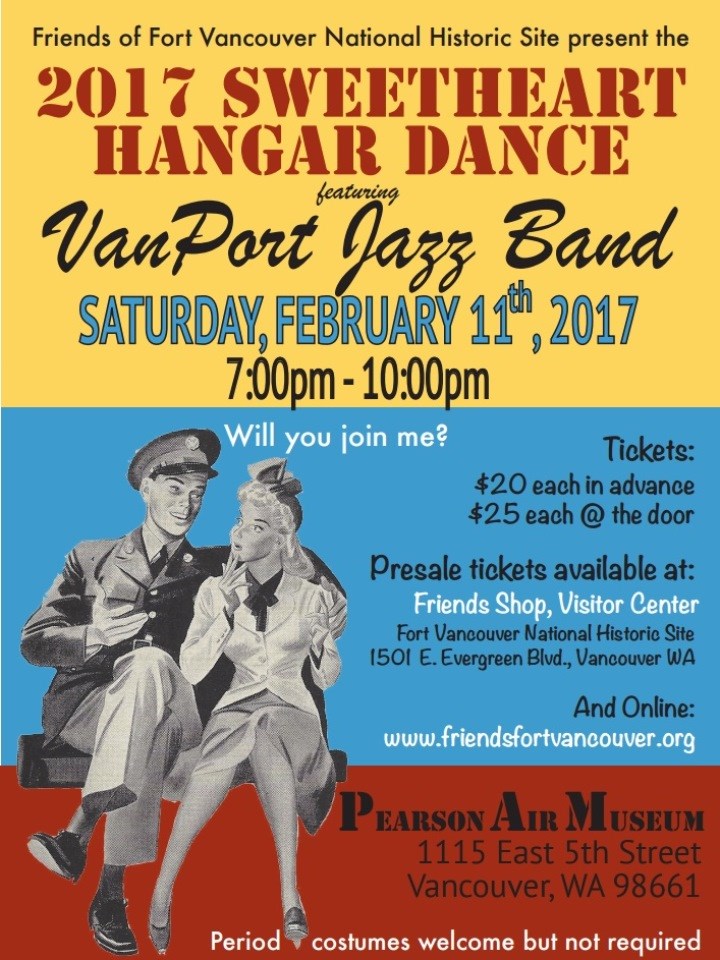The event poster, set against a vibrant yellow backdrop with a bold mix of red, black, and blue text, is an illustration highlighting a charming scene. In the foreground, a couple is seated on a bench, exuding a vintage feel; the man, dressed in a full military uniform complete with cap, jacket, and pants, has his hands tenderly resting on the woman’s shoulders as they look into each other’s eyes. The woman is attired in a blouse and skirt combination, complementing the nostalgic theme. 

The poster advertises the 2017 Sweetheart Hanger Dance, presented by Friends of Fort Vancouver National Historic Site. The event, featuring the Vanport Jazz Band, is scheduled for Saturday, February 11th, 2017, from 7 PM to 10 PM. An inviting message on the poster reads, "Will you join me?" in white text against a blue backdrop. Ticket prices are listed as $20 in advance and $25 at the door, with pre-sale tickets available at the French Shore Visitor Centre. The event venue is the Pearson Air Museum, located at 1115 East 5th Street, Vancouver, WA 98661. The poster also mentions that costumes are welcome but not required, completing the festive and nostalgic appeal of the event.